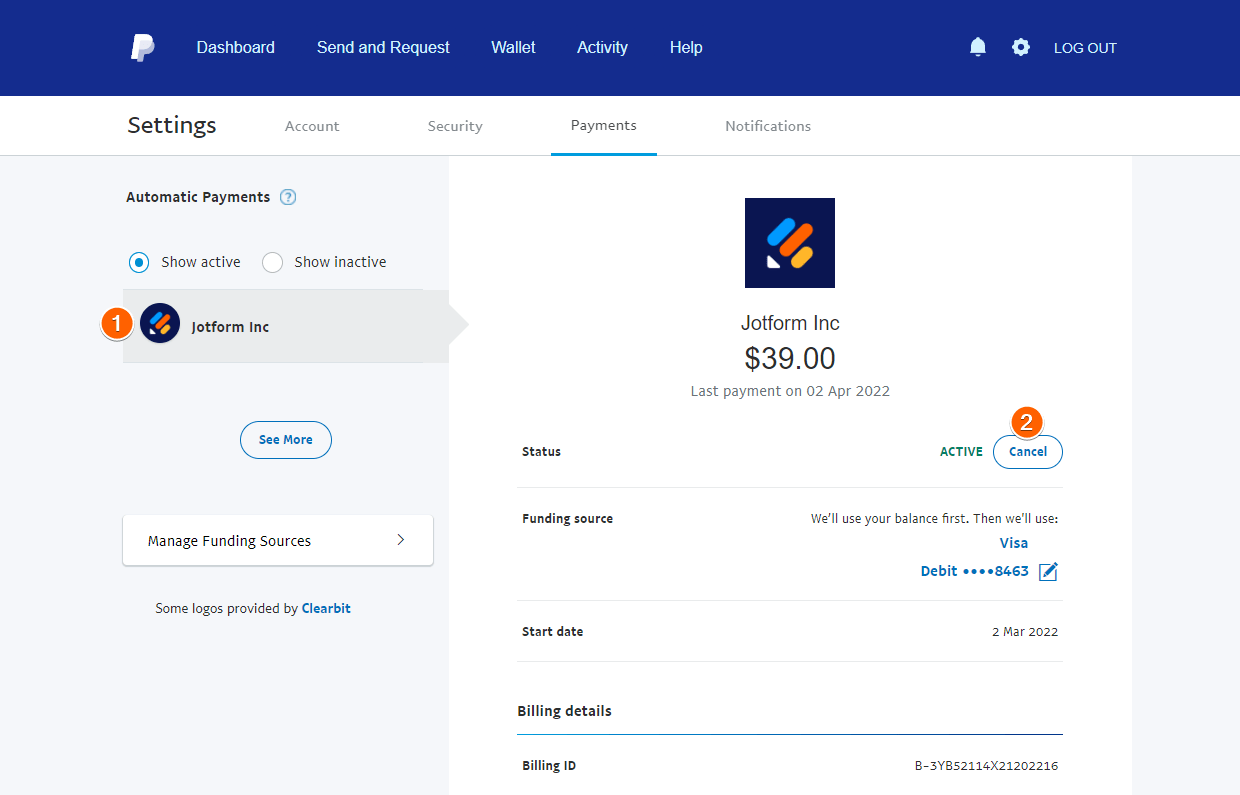This screenshot captures the PayPal website's interface after a user has logged in. At the top, a blue banner displays the PayPal logo—a white 'P' with a shadow effect—positioned on the far left. The navigation bar includes options in white or light blue text: Dashboard, Send and Request, Wallet, Activity, and Help. Further to the right, icons for notifications (a bell), settings (a gear), and the words LOGOUT in all caps are also visible.

Below this, there is a secondary navigation menu. Here, Settings is bolded, indicating that the user is currently on the Settings screen. Other available but not bolded options within this menu are Account, Security, Payments, and Notifications. 

The focus is on the Payments section within Settings, specifically concerning JotForm, Inc. The interface indicates automatic payments to JotForm, Inc., with an active status. The payment amount listed is $39, last paid on April 2, 2022, with an option provided to cancel this automatic payment.